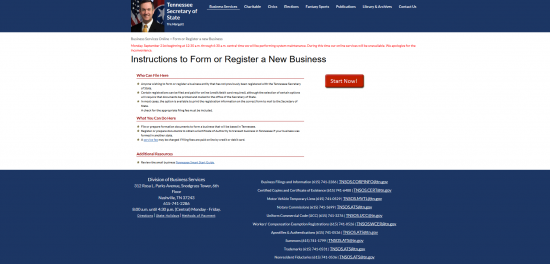A screenshot of a webpage featuring a dark blue bezel dominates the image. An individual dressed in a black tuxedo with short black hair stands next to an American flag, holding a gold trolley. On the right-hand side, white text reads "Tennessee Secretary of State." Underneath, an informational section details "Instructions to Form or Register a New Business." Adjacent to the individual, there are eight small tabs, though their text remains unreadable even upon zooming in. Below the main instruction header, red subheaders and cautionary red text are visible. A prominent red rectangular button with white text is positioned to the right of the instructions. Both the left and right sides of the large blue bezel at the bottom of the page display more white text, though the specific details are blurred. The majority of the background between the blue bezels is white, making the central elements stand out clearly.